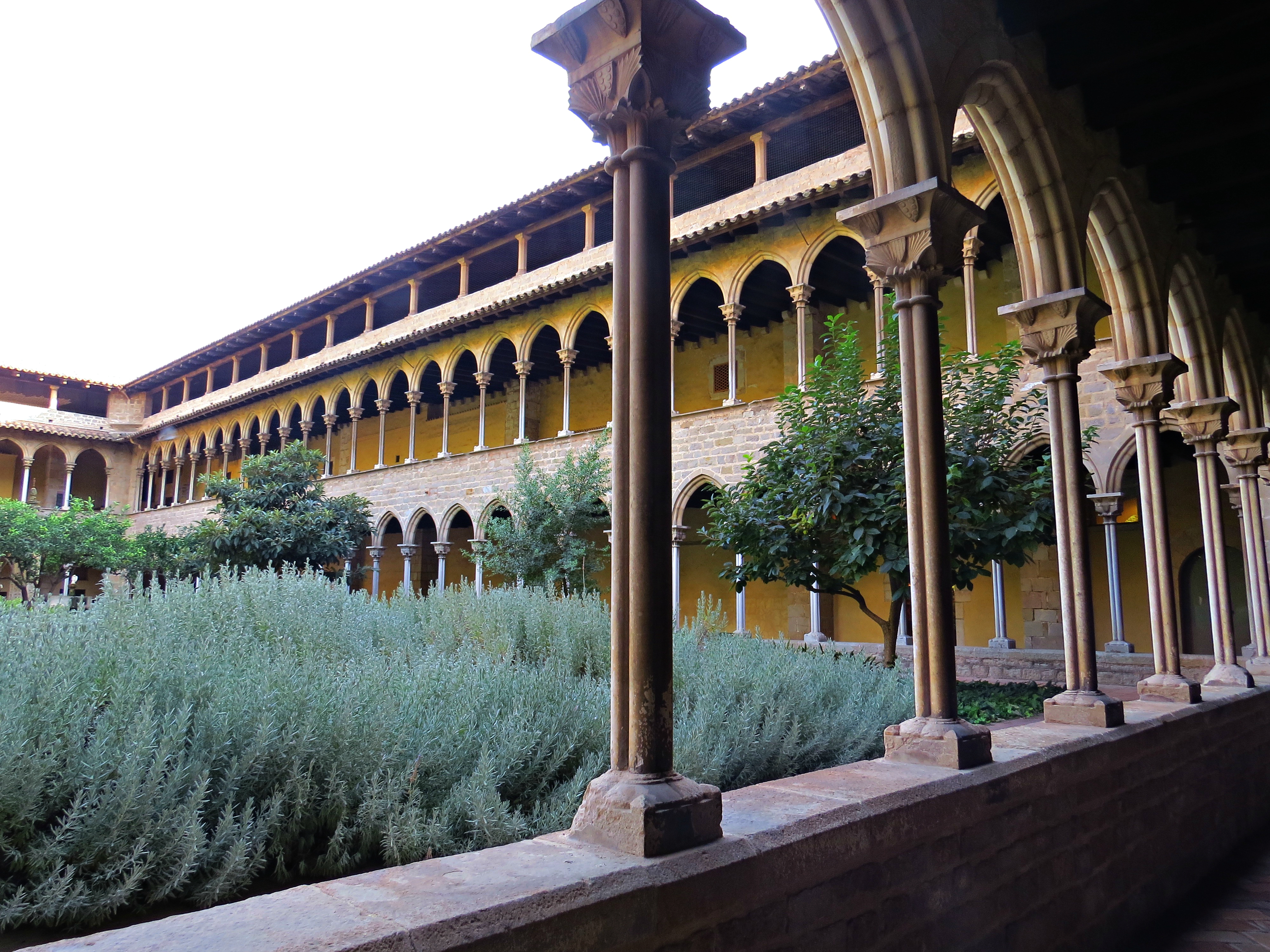This photograph features a beautiful, symmetrical courtyard encircled by a large, U-shaped building that appears to be a very nice hotel or similar structure. The building showcases an elegant design with abundant arched columns supporting covered walkways on two identical lower levels. These levels feature long patios beside the courtyard, while the top level has vertical columns instead of arches, giving it a slightly different appearance. The arched hallways and patios are bordered by numerous beams, brickwork, and marble statues, all contributing to the grandeur of the scene. Yellow-hued walls and a tiled roof add to the architectural charm. The courtyard itself is lush, filled with grass, some small fruit trees, and light green shrubbery. A white sky looms overhead, and there are lights mounted on the building walls, but no rain gutters, meaning rain would fall directly to the courtyard's greenery. The entire scene is devoid of people, allowing the focus to remain on the intricate and symmetrical design of the courtyard and building.